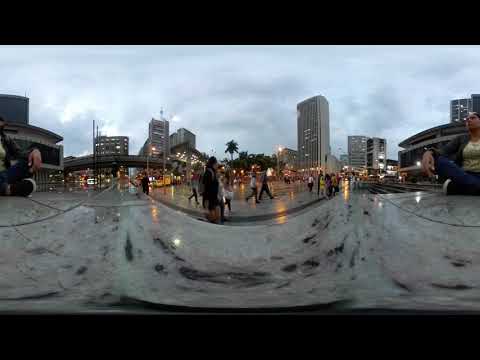This image is a detailed 360-degree panoramic view of an outdoor urban scene, taken with a fisheye lens. The photograph captures a bustling city atmosphere on a rainy, overcast day. The gray sky is filled with blue and white clouds, giving a nuanced texture to the atmosphere. The wet streets and sidewalks glisten from the rain, reflecting numerous city lights, both white and yellow.

Prominently featured is a person sitting cross-legged on black and white tiled pavement wearing a yellowish-beige blouse, a long-sleeve sweater, blue jeans, and sneakers. Her dark hair frames her face as she becomes a focal point amid the busy backdrop. 

The scene is filled with various elements, including a mixture of skyscrapers, some of which illuminate with lights, and smaller buildings directly behind the seated woman. There are palm trees scattered between the buildings, bringing a touch of greenery to the urban landscape. In the distance, a large stadium-like structure and a bridge-like feature contribute to the complexity of the scene. The overall ambience suggests dusk, as artificial lights begin to dominate, highlighting the vibrancy and activity of the city despite the rainy conditions. The image has black borders at the top and bottom, framing this dynamic city snapshot.